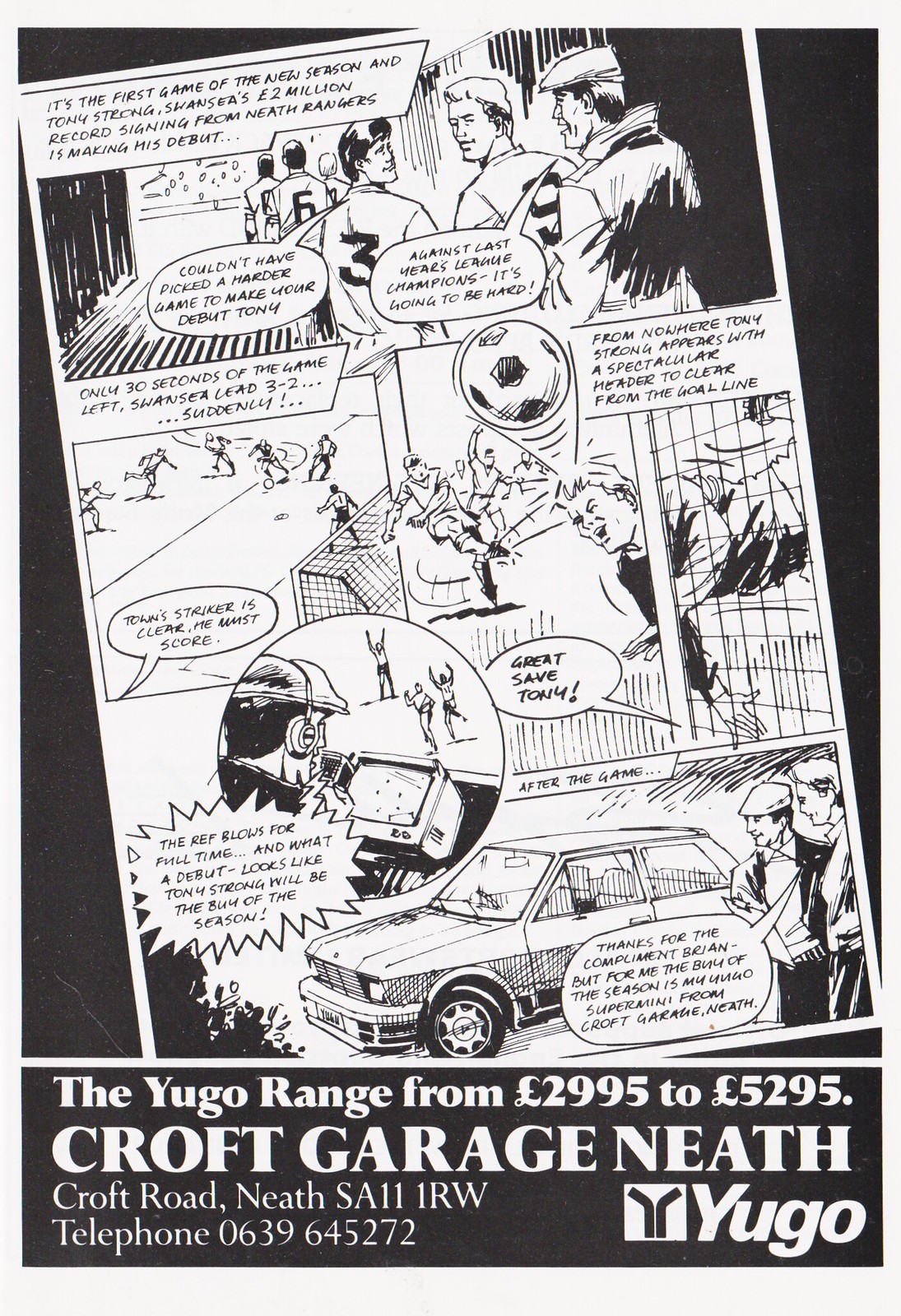This is a detailed black-and-white photo of a soccer-themed comic strip with an advertisement for a car at the bottom. The comic strip narrates the debut of Tony Strong, a record signing for Swansea, in the first game of the new season against last year's league champions. The strip highlights conversations between players about the toughness of the game and builds up to a climactic moment where Tony, the goalie, makes a crucial save, leading Swansea to a 3-2 victory. 

The layout of the comic includes various action shots of soccer players with text bubbles depicting their dialogues. Above, there's an image of players in conversation, and in the central section, there are two images showcasing the game action. At the bottom, aside from additional comic text, there is a depicted image of a car with two individuals looking at it.

The advertisement below the comic strip features the Yugo car range, priced from 2,995 to 5,295 euros. It provides details of the Croft Garage located in Neath, with the address Croft Road, Neath, SA111RW, and the contact number 0639-645272. The text of the advertisement is in white on a black background, contrasting the overall black-and-white comic. The Yugo logo appears at the bottom right of the advertisement. The entire piece appears to be a mix of hand-drawn artistry and digital composition.